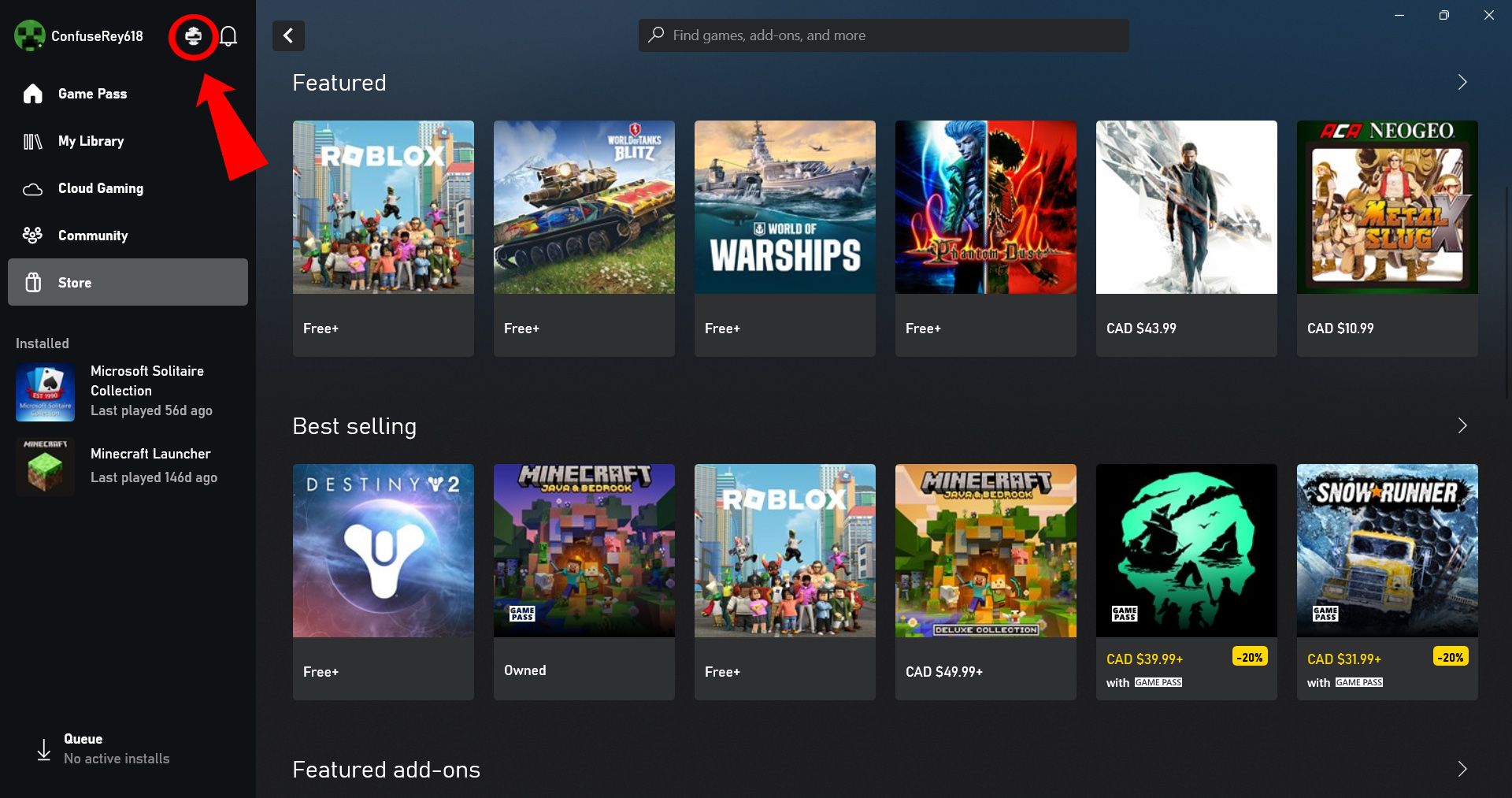In the image, the left-hand side features a column with several menu options and game titles. At the top of the column, there is a section labeled "Compute" with a RAID 618 indicator. Below that, a red circle icon and a bell symbol are displayed. The column lists categories including Game Pass, My Library, Cloud Gaming, Community, Store, Install, Microsoft's LTE Collection, Let's Play Physics, and History of Minecraft. Several game titles are mentioned: "Minecraft Launcher," which was played about 6 days ago, "Roblox," "Will the Things Plays," "World of Warships," "Phantom Dust," "Quantum Brain," "Cinebench Linux," and "Destiny 2." Multiple versions of Minecraft—Java, Bedrock, and Deluxe Collection—are also visible. To the right of the column, the "Sea of Thieves" icon is prominently displayed. Additionally, the game "SnowRunner," featuring a truck navigating through snowy terrain, can be seen.